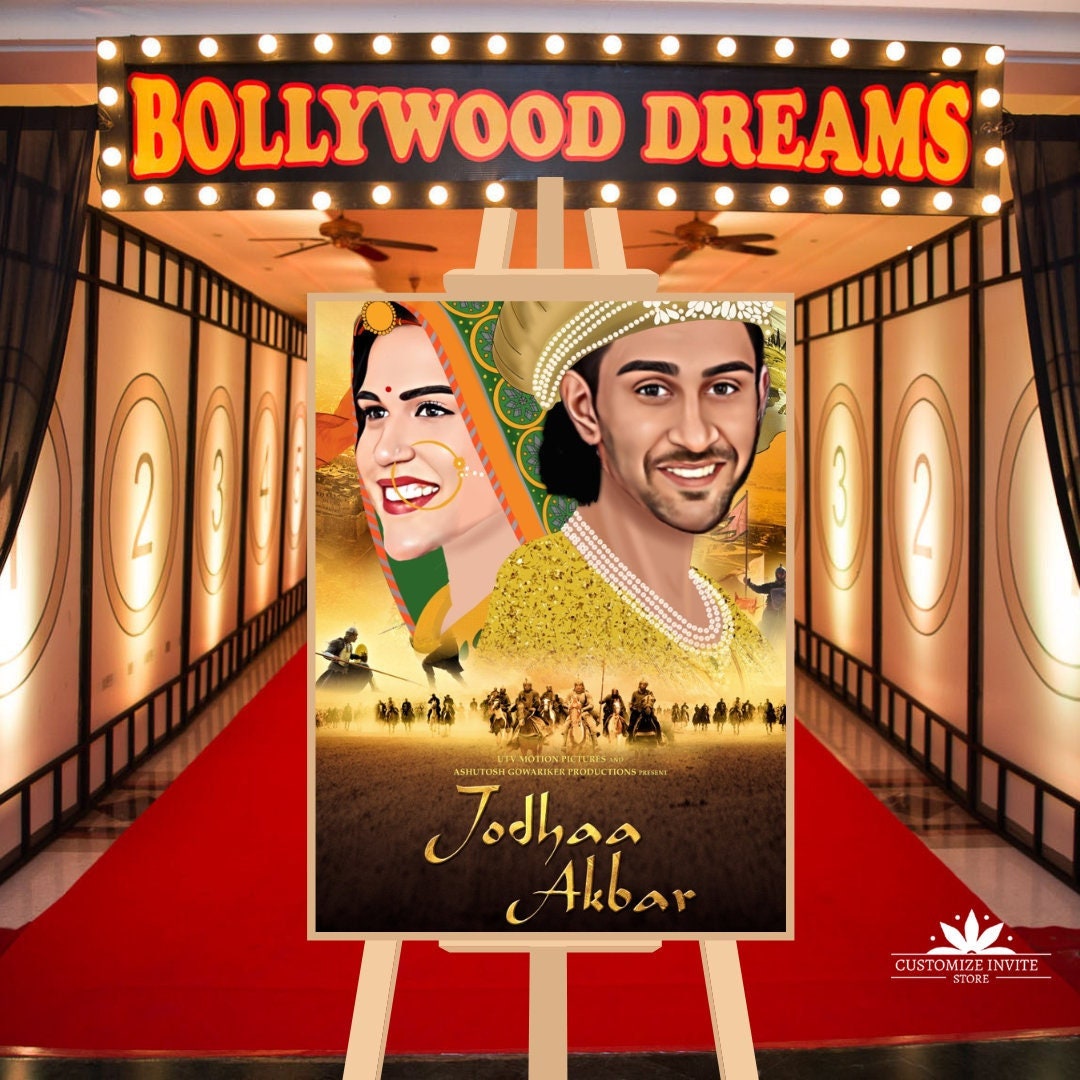The image depicts a vibrant advertisement for a Bollywood movie titled "Jodha Akbar." At the top, a black banner with yellow font outlined in red reads "Bollywood Dreams," and the banner is adorned with round movie theater lights reminiscent of classic cinema marquees. Below it, an easel holds a prominent movie poster. Featured on the poster are an elaborately dressed man and woman. The woman wears a green headscarf adorned with yellow circles and an orange border, complemented by a large gold nose ring and a bindi dot. The man, clad in regal gold attire, dons a sequined turban and multiple strands of pearls around his neck. Beneath the duo, a row of warriors on horseback is depicted, exuding a sense of epic grandeur. The movie title "Jodha Akbar" is prominently displayed in the lower right corner of the poster, while a caption at the bottom reads "Customite Invite Store." The setting appears to be a movie theater hallway with a red carpet and numerical markers on the walls, enhancing the nostalgic cinematic ambiance.